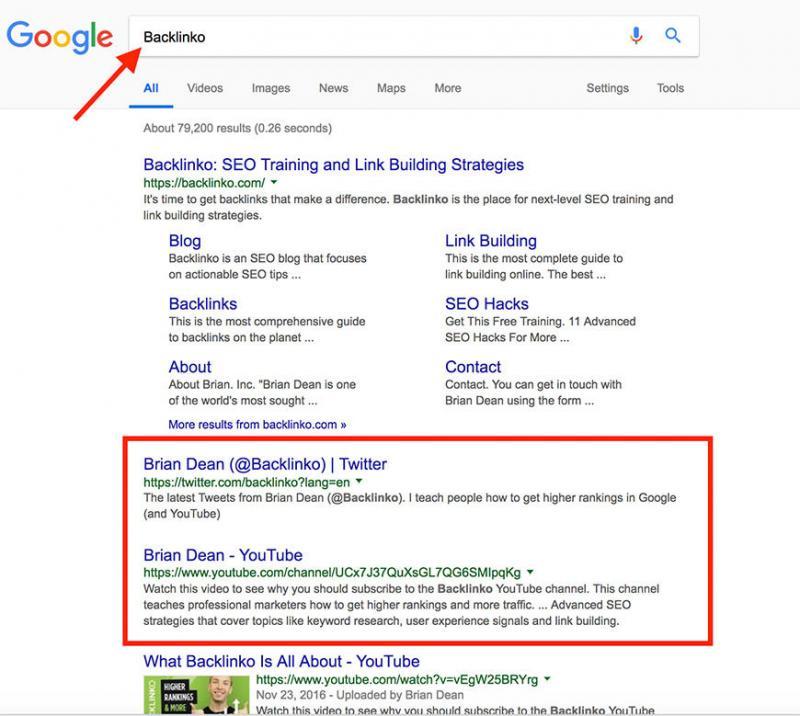This cropped screenshot depicts a Google search page. In the top-left corner, the iconic Google logo is visible. Adjacent to the logo on the right, the search bar prominently displays the query "Backlinko." A noticeable red arrow, digitally added to the image, diagonally points to the word "Backlinko" within the search box.

At the bottom of the search results, there is an edited red box highlighting key search entries. The first highlighted result reads "Backlinko Brian Dean," accompanied by the social media handle @backlinko from Twitter. The second highlighted result within the red box indicates Brian Dean's YouTube channel. The background of the web results is predominantly white, accentuating the red arrow and box that guide the viewer's attention to the typed search term and its corresponding results.